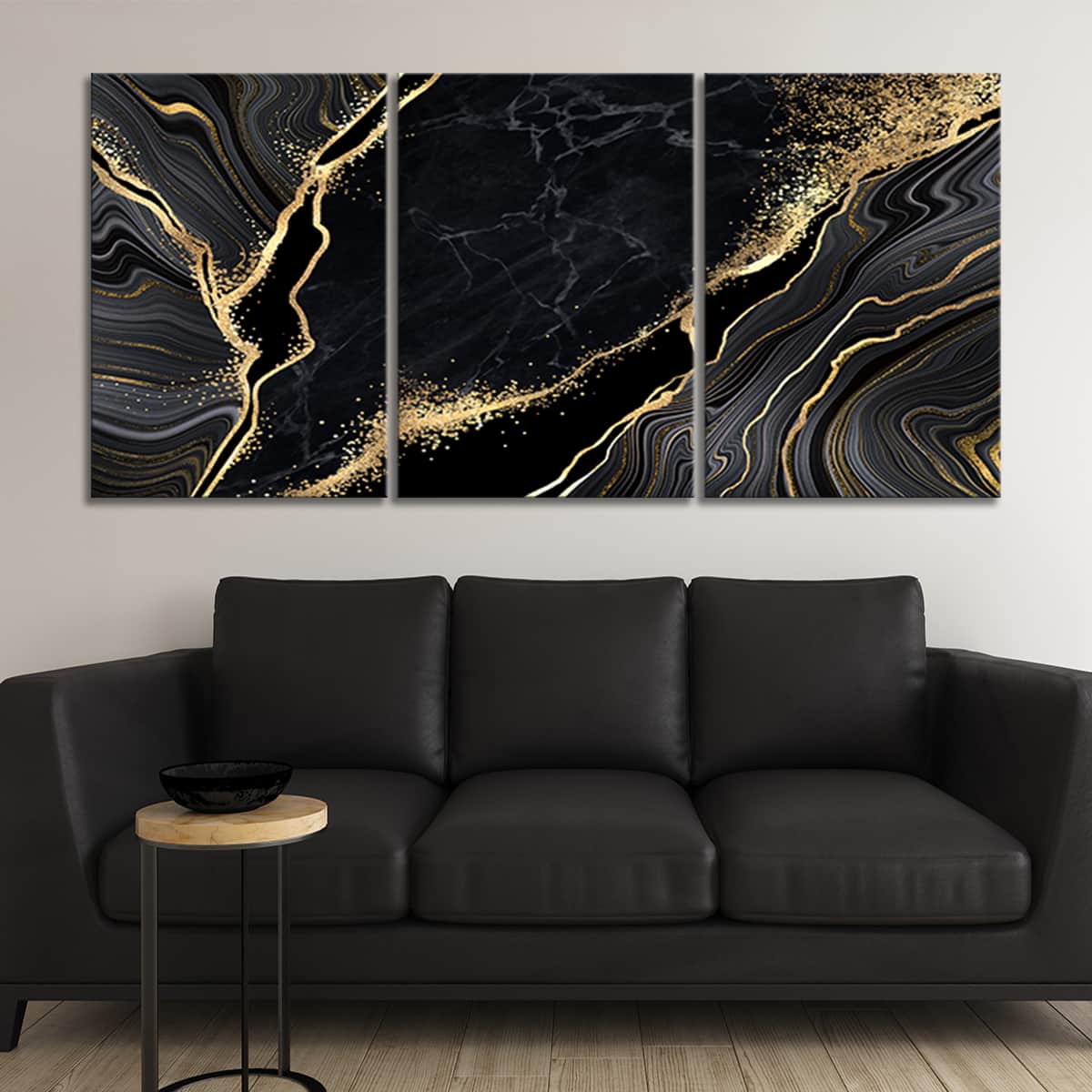This indoor color photograph features a three-seater black couch with a slight sheen, characterized by three bottom cushions, three back cushions, and squared arms, lending it a squared overall look. The couch, possibly made of fabric or leather, rests on a light-colored wood-paneled floor. In front of the couch stands a small wooden circular table with black metal legs, topped with a black bowl. The backdrop is a white or gray wall adorned with a striking trio of black and gold abstract canvas paintings, each separated by fine borders. The dynamic art pieces display sweeping golden strands and white details, resembling a geode’s intricate patterns, with a notable Y-shaped gold spatter in the leftmost piece.